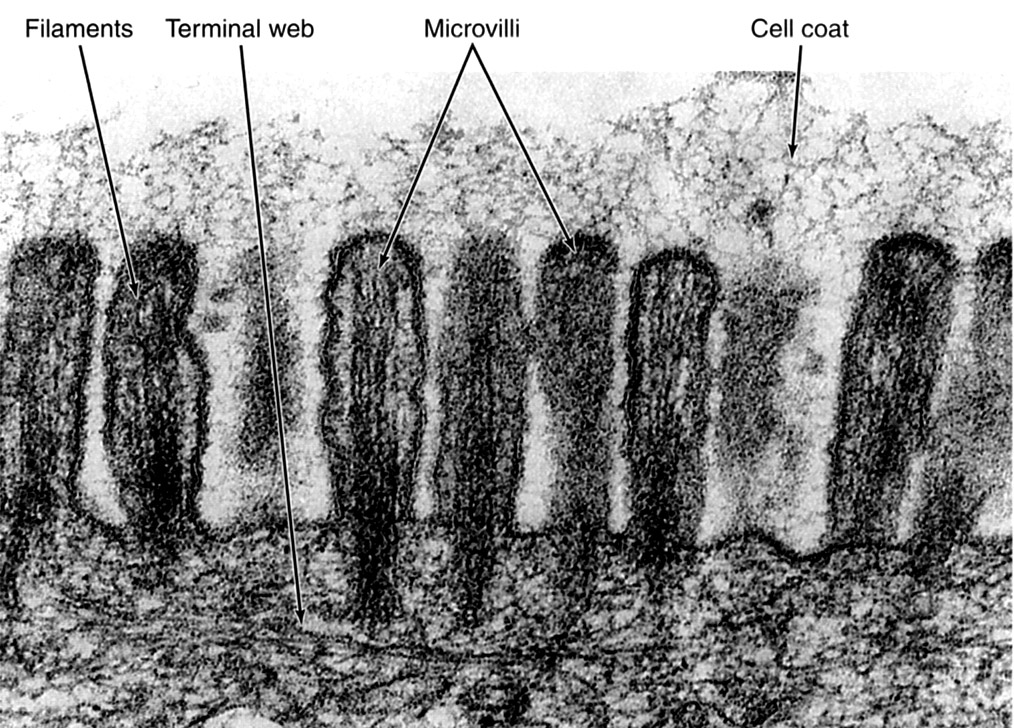This black and white diagram, resembling a grainy microscope photograph or a highly detailed illustration, depicts cellular structures and their components. At the top, set against a white background, labels and arrows identify different parts of the cell. The term "filaments" points to black, elongated, finger-like projections on the far left, while "terminal web" highlights a dense, crayon-outlined region at the bottom, resembling rough, gravelly ground or an interwoven mesh. To the right of "filaments," the term "microvilli" marks additional black columns extending upwards. These projections are capped by a lighter, greyish mesh, described as the "cell coat," providing a contrasting background. The overall image is gray and blurry, with black structures crisply standing out against a lighter gray backdrop. This intricate depiction of cell components suggests a closer look at cellular microstructures and their interactions, though the absence of color and the abstract presentation make it somewhat challenging to discern specific details.